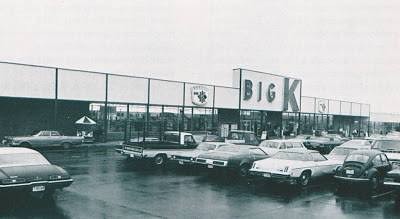The image is a black and white photograph depicting the parking lot of a store labeled "Big K." The exterior of the store is painted white and features rectangular architectural elements with the store's name, "Big K," prominently displayed in bold letters. The scene appears to date back to the late 1970s, as evidenced by the presence of bulky cars typical of that era. Notably, a dark-colored Volkswagen Beetle is parked among the rows of vehicles. Although the parking lot lines are not visible upon close inspection, the photograph clearly shows multiple rows of parked cars, adding to the nostalgic ambiance of the setting.